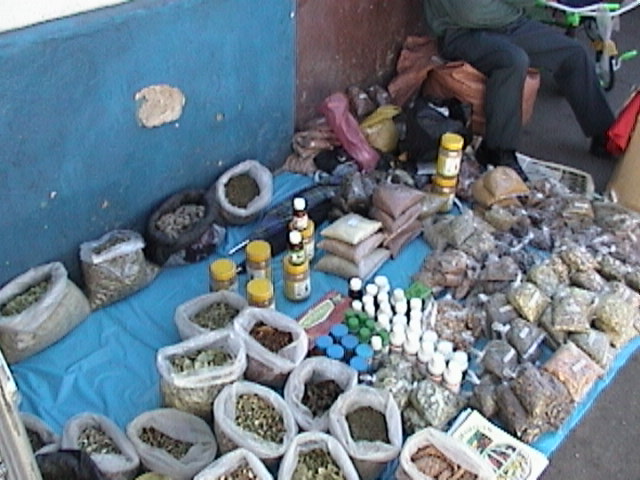The image depicts a street vendor selling an assortment of products on a concrete sidewalk covered by a light blue plastic tarp. Lined up on the tarp from the bottom left corner to the center are numerous white, semi-transparent plastic bags arranged in circular rows. Each bag appears to contain various types of grains, spices, or dried goods. Some bags are open, displaying their contents, while others are sealed and labeled with white tags. Additionally, several jars and pre-packed clear bags are neatly arranged for sale.

The vendor is seated on a brown sack next to his merchandise. He is dressed in black slacks, black shoes, and a green shirt, though his face is not visible as it is cropped out of the shot. Behind him is a wall, predominantly painted blue, with a conspicuous white patch where the plaster has chipped off, revealing the concrete underneath. The photograph is a wide vertical shot, focusing on the items for sale against the backdrop of the street and wall.